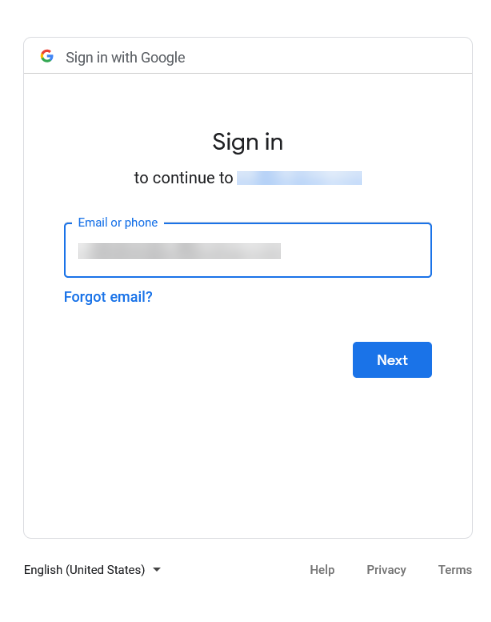A detailed caption for the image could be:

----

"This image depicts the Google account sign-in page. At the top, there is a header featuring the Google logo alongside the text 'Sign in with Google'. Below this, there's a prompt stating 'Sign in to continue to', with the specific service or website obscured. The primary area of the page includes a text box labeled 'Email or phone number', where users should enter their login credentials. Beneath this field, there is a 'Forgot email?' link which can be used to recover the associated email address for the account. Following the input field is the 'Next' button, colored blue with white lettering, which navigates the user to the password entry phase of the login process after they've entered their email or phone number. The bottom section of the page allows users to select their preferred language, which in this instance is set to English (United States). In the lower right corner, there are links for 'Help', 'Privacy', and 'Terms'. The 'Help' link provides assistance and support, potentially redirecting users to contact Google support for issues beyond password recovery."

-----

This revised caption provides a clear, detailed description of the elements present on the Google sign-in page, ensuring it is comprehensive for users who are not viewing the image.